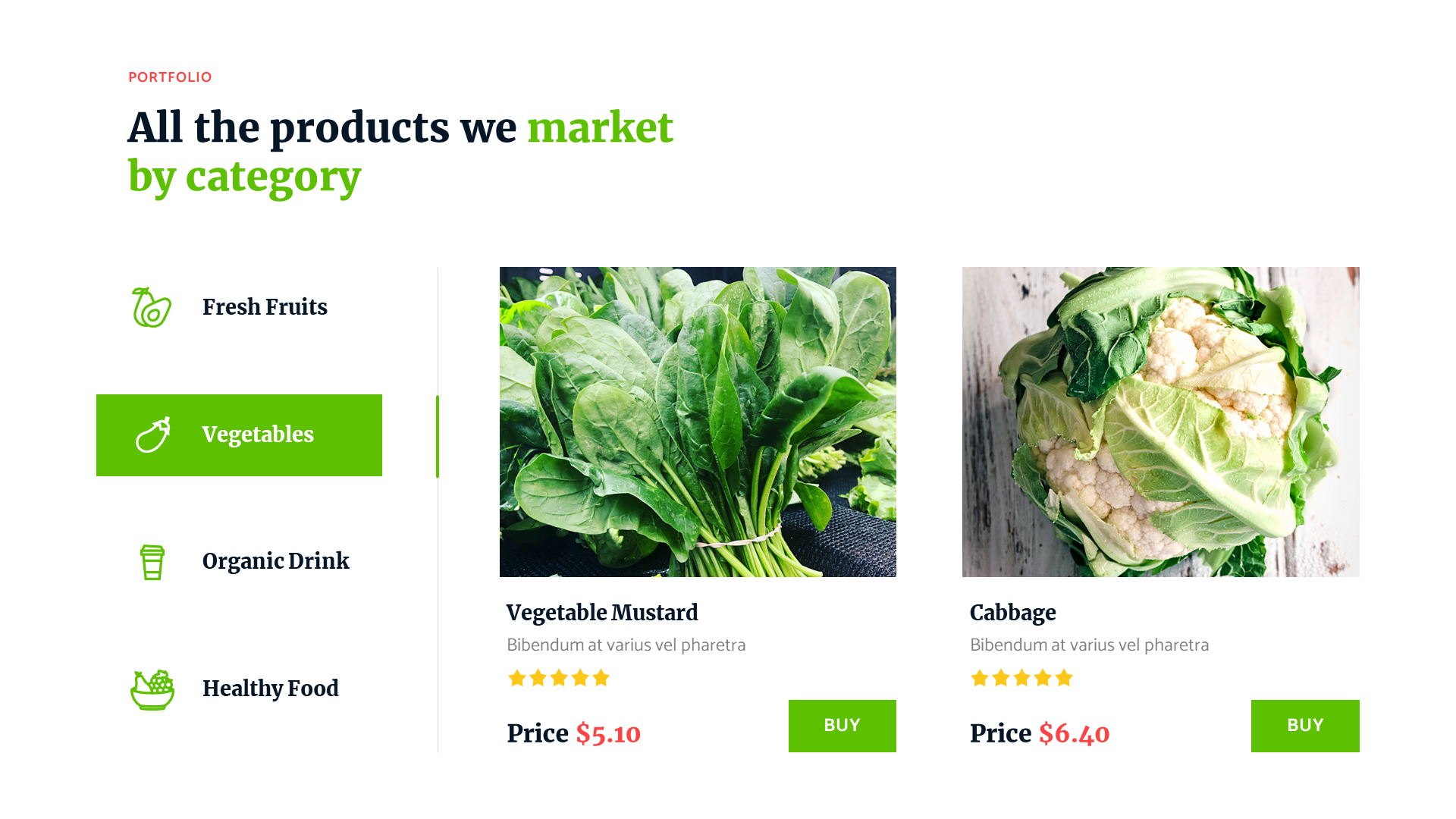The web page screen capture prominently features a well-organized portfolio of products, categorized clearly for easy browsing. At the upper left corner, the word "Portfolio" is prominently displayed in red text. Directly beneath, a descriptive label in black and green text reads, "All the products we market by category." A navigational frame below this label lists product categories in black and green: "Fresh Fruits," "Vegetables" (highlighted in green), "Organic Drink," and "Healthy Food."

Central to the image is a picture of vibrant, green mustard leaves set against a neutral gray background. Underneath the image, the product name "Vegetable Mustard" is written in bold black text. Directly below the product name, the rating is displayed with five yellow stars, indicating high customer satisfaction, and the price is marked clearly in black and red text: "Price $5.10." At the bottom of this section, a green "Buy" button invites customers to make a purchase.

To the right side of the central image, an additional image of a fresh, leafy cabbage is visible, providing another example of the website's visual layout and product offering.